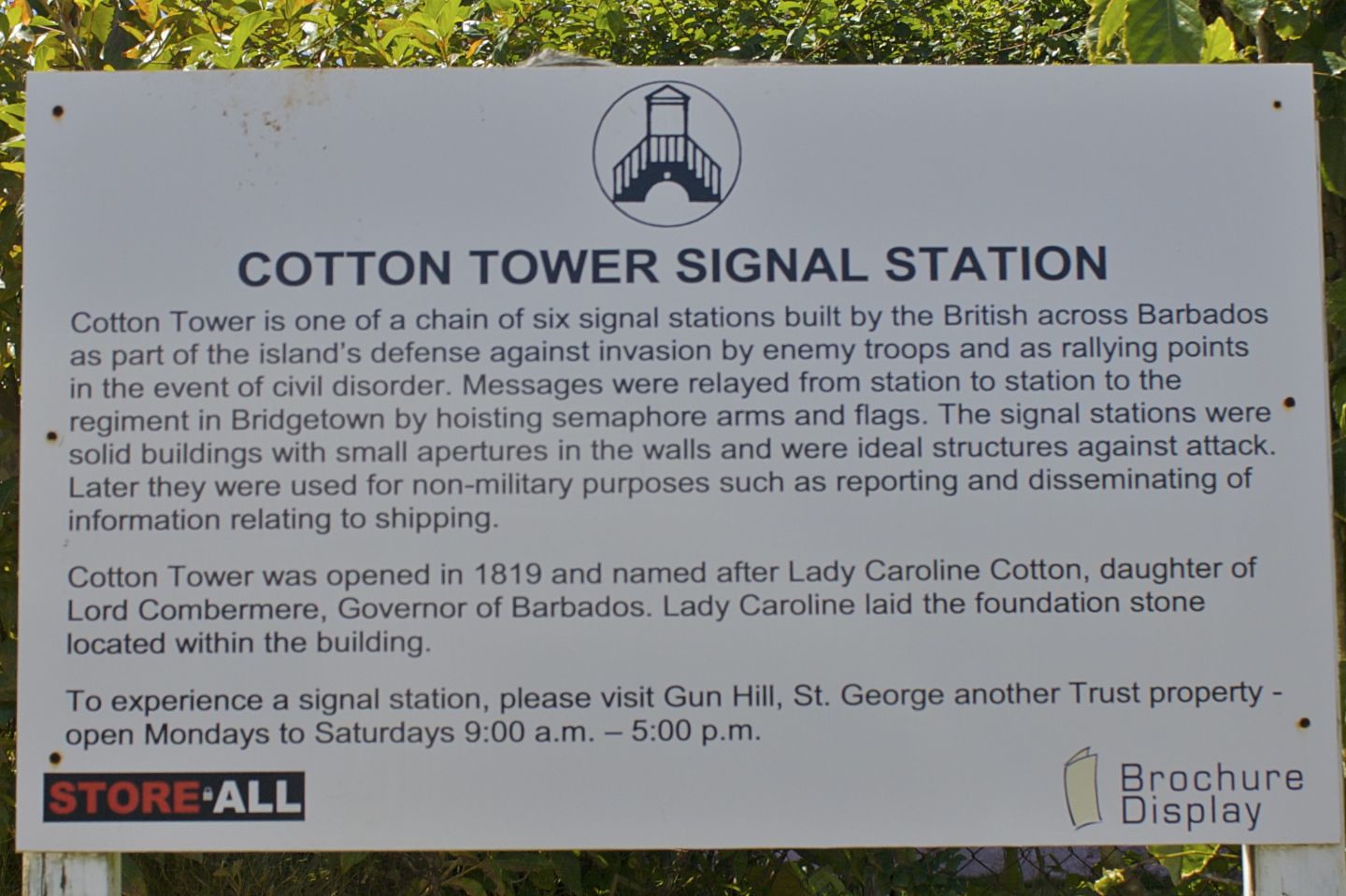The image is a color photograph of a sign mounted on two poles, positioned outside against a backdrop of green leaves. The sign has a white background with a dark circular image of a signal tower at the top center. Below the image, the text reads "Cotton Tower Signal Station." The sign provides detailed historical information, stating that Cotton Tower is part of a chain of six signal stations built by the British across Barbados as a defense mechanism against enemy invasion and as rallying points during civil disorder. These stations communicated by relaying messages through semaphore arms and flags to Bridgetown. Constructed as solid buildings with small apertures in the walls, they were well-suited to withstand attacks. Later, they served non-military purposes like reporting and sharing shipping information. Cotton Tower, opened in 1819, was named after Lady Caroline Cotton, daughter of Lord Combermere, Governor of Barbados, who laid the foundation stone located within the building. Visitors can experience this historical site by visiting Gun Hill, St. George, and other trust properties, open Mondays to Saturdays from 9 a.m. to 5 p.m. At the bottom of the sign, there are indicators for a "store all" section on the left and a "brochure display" on the right.